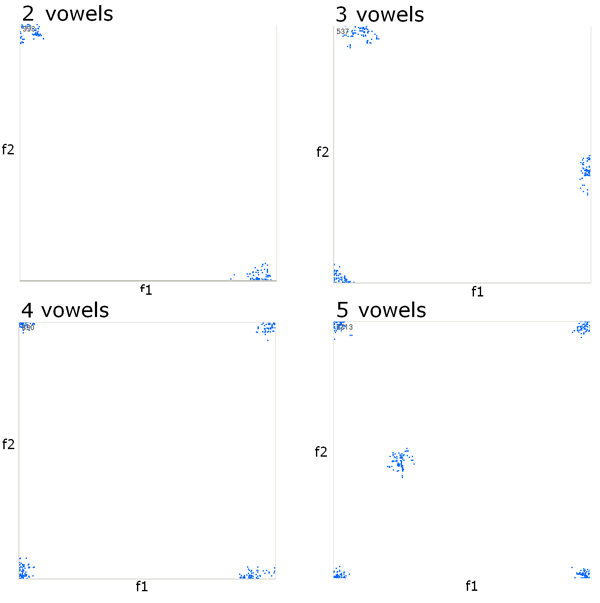In this image, we see a completely white background with four distinct boxes arranged in a windowpane style format. Each box contains a dotted line graph representing auditory levels, with varying numbers of vowels as indicated by the titles: the top left box is labeled "two vowels," the top right "three vowels," the bottom left "four vowels," and the bottom right "five vowels." Along the X-axis of each graph is labeled "F1," and the Y-axis is labeled "F2." The dotted lines appear to cluster predominantly around the upper sections of the Y-axis and the far right of the X-axis. The image also includes some blue splotches scattered across the background, adding a hint of color to the predominantly black, white, and blue theme. The organized layout and educational content suggest that this image is designed for instructional purposes, possibly from a school workbook or classroom material.